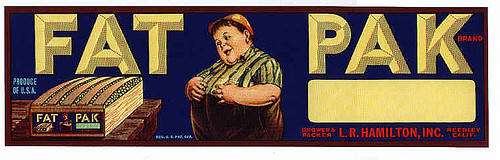This advertisement features a nostalgic, vintage-inspired design, though it’s uncertain if it’s genuinely old or a modern creation with a retro aesthetic. The layout is a horizontal rectangle framed with a brown edge, mimicking an old-fashioned frame. The background is a deep blue, providing a striking contrast to the central elements.

Prominently displayed in tan, shadowed, large capital letters, the brand name "FAT SPACE PACK" catches the eye. On the left-hand side, the phrase "Produce of USA" further emphasizes the product's origin. 

Centrally located in the image is a substantial wooden box, set upon a rough, rustic wooden table surface. The box appears to contain peas, and its end prominently features the same "FAT SPACE PACK" label described earlier.

In the heart of the composition stands a notably chubby boy. He is dressed in oversized brown pants and a green and tan striped shirt. Sporting a double chin, an orange cap atop his brown hair, he gazes intently at the box of peas. 

To the right of the image, additional details about the product's origin can be found: the text "Growth and Packer" followed by "L.R. Hamilton, Incorporated, Wheatley, California." These details provide authenticity and a touch of personalized history to the advertisement.